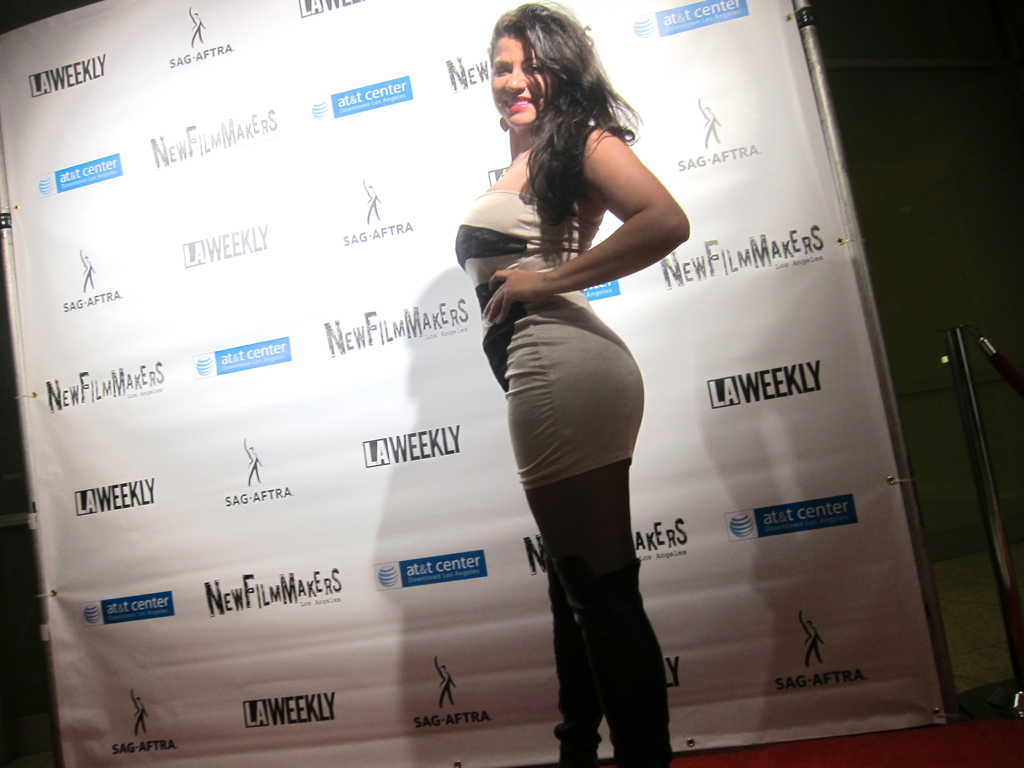In this vibrant image, a striking woman is prominently positioned at the center, exuding confidence and elegance. She has dark hair cascading over her left shoulder and is adorned with eye-catching red lipstick that adds a bold touch to her look. Dressed in a tight black and gray striped dress that accentuates her curvaceous figure, she wears high black boots that enhance her modern, fashionable appearance. The dress, a stylish short skirt leaving her shoulders and upper chest bare, complements her sophisticated aura. 

She stands laterally on what seems to be a red carpet or stage backdrop, with a large poster behind her showcasing various iconic logos and ads in black and white, including LA Weekly, SAG-AFTRA, AT&T Center, and New Filmmakers. These logos are scattered across the white background, adding a subtle contrast with some shadows enhancing the overall composition. The setting appears to be indoors, likely at an award show, contributing to the glamorous atmosphere of the scene. The overall color palette predominantly features black, white, and blue, with splashes of pink from her lipstick and a few other accent colors, adding to the modern and chic design aesthetic of the image.